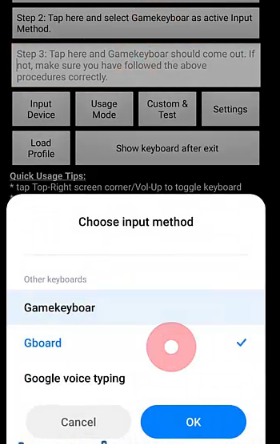In this screenshot, we see a settings interface on a smartphone. The upper section of the image displays the "Choose Input Method" menu. This menu presents three keyboard options: "Game Keyboard," "Gboard," and "Google Voice Typing," with "Gboard" highlighted in blue as the selected choice. Below this selection, there is a large blue button labeled "OK" and a smaller light gray button labeled "Cancel" to its left.

The background of the menu is predominantly white, creating a clear and easily readable display, with black text inside the blue and gray buttons and white text at the bottom. Moving further down the image, the background transitions to black and contains gray text boxes with small black text inside them. These sections provide detailed step-by-step instructions for activating or changing the input method.

The image as a whole is a tall rectangle, oriented vertically, and also features additional buttons for settings, usage mode, and input device configurations.